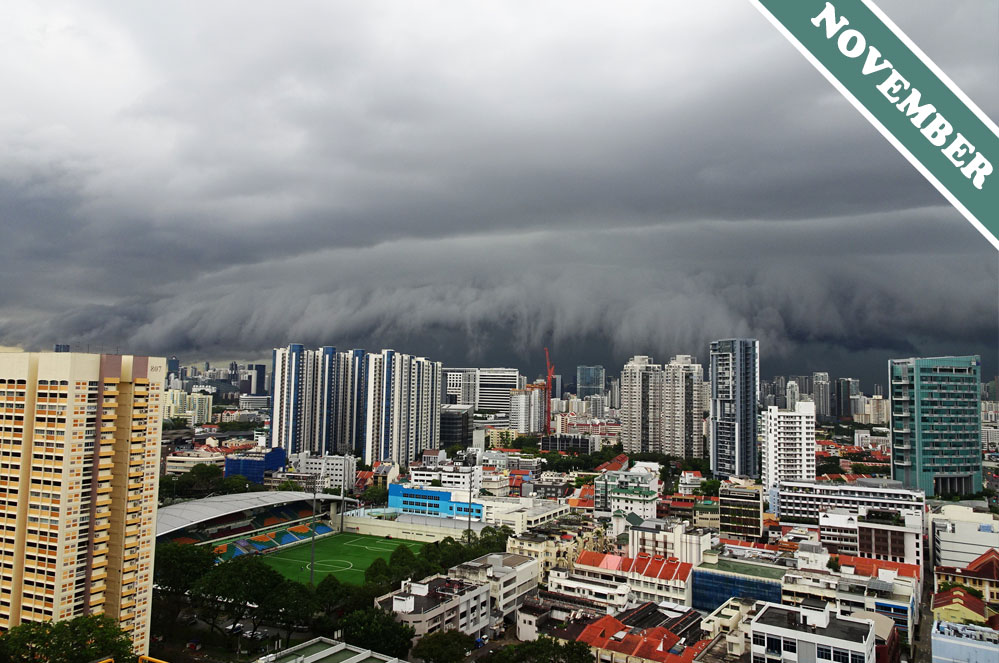This detailed photograph captures an industrial scene of a large city under ominous, stormy weather. The sky, filled with dark, gray clouds, looms heavily over the cityscape, almost resembling a massive wave about to engulf the urban area. In the top right corner of the image, a green and white diagonal banner reads "November," suggesting it might be the cover for a calendar. 

The city is composed of a variety of buildings of different sizes and colors, painting a diverse urban landscape. On the left side of the photograph, a tall beige building, possibly an apartment complex or a hotel, stands prominently. This building features some brown spots and contrasts with the surrounding gray office buildings positioned behind it. Towards the right side of the foreground, buildings with distinctive red roofs are visible, along with smaller structures that add to the city's architectural variety.

A notable element in the scene is a large football stadium with a green, open field nestled towards the lower middle of the image. The stadium is outlined by trees, providing a touch of greenery amidst the industrial setting. The juxtaposition of the stadium with the surrounding skyscrapers highlights the scale and height of the clouds, which seem poised to overtake the city imminently.

Overall, this image powerfully conveys a city bracing for a severe weather event, with the dramatic storm clouds creating an atmosphere of impending doom and destruction.